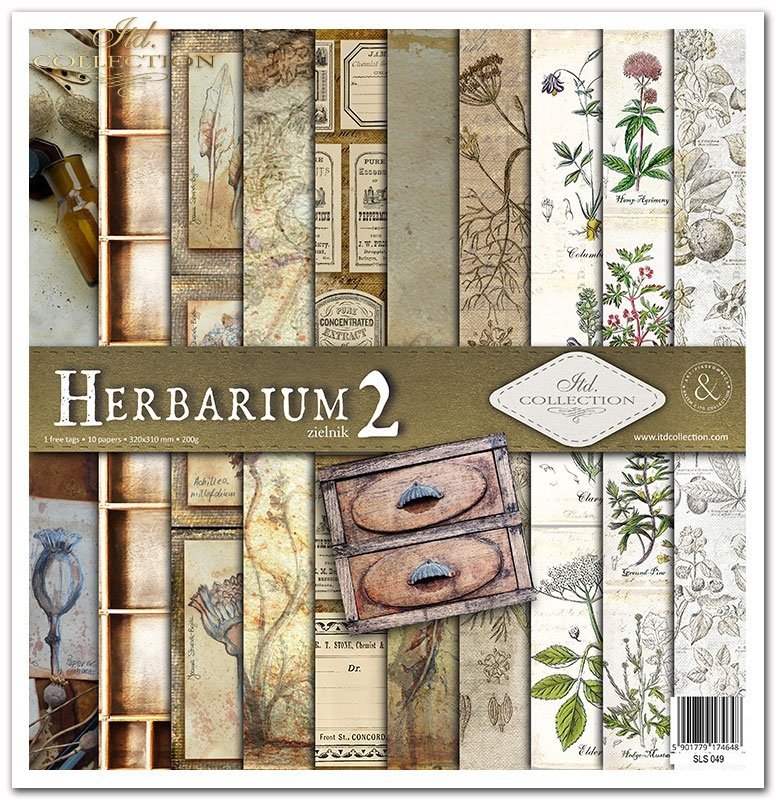The image depicts the cover of a set of scrapbook papers titled "Herbarium 2," presented in a white font. The cover, designed to appear as if showcasing the spines of long, thin books arranged in a row, suggests a vintage collection theme. The right side features "Limited Collection" inside a diamond shape, alongside a logo with an ampersand encircled by unreadable text. Below this, the URL "www.itdcollection.com" is printed in a light font. Additionally, there is a barcode at the bottom right corner, labeled 901779174648, with "SLS049" beneath it. The scrapbook papers inside feature designs reminiscent of antique botanical illustrations, vintage pharmacy labels, and medical illustrations. The cover visually mimics ten book spines with varying antiquity prints, predominantly showcasing flowers, leaves, and other plant-related motifs, giving a rich, historical aesthetic.